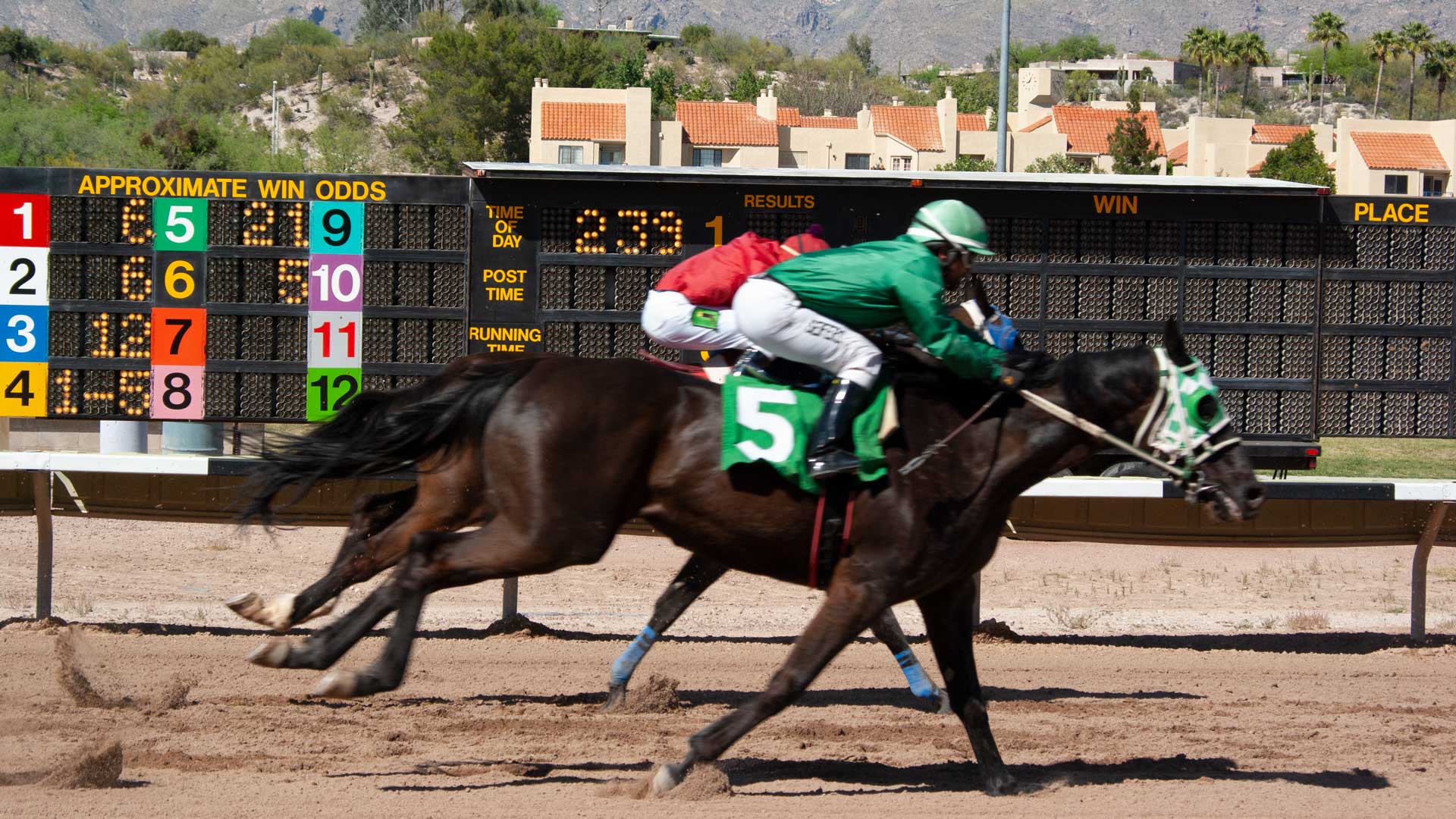In this vivid and dynamic photograph of a horse race, two dark brown horses with their jockeys are captured mid-stride on a sunlit track, racing toward the right side of the frame. The jockey in the foreground is clad in a green jacket, green hat, and white pants, riding horse number five, identifiable by the green number plate attached to the horse's harness. The horse wears a specialized mask to maintain its focus. Slightly behind, another jockey dressed in a red jacket, red hat, and white pants rides a similarly colored horse. Both horses are glistening in the bright sunlight, showcasing their sleek coats and intense speed.

In the background, visible behind the race track, is a scoreboard displaying approximate win odds: with horse number one and number two both having a one-sixth chance of winning, horse number three with a one-twelfth chance, horse number four with a one-fifth chance, horse number five with a one-twenty-first chance, and horse number six with a one-fifth chance. The scene also includes additional boards showing real-time race results and timings. Adding to the picturesque setting are distant houses with terracotta roofs, palm trees, and mountains, suggesting the location might be in Southern California.